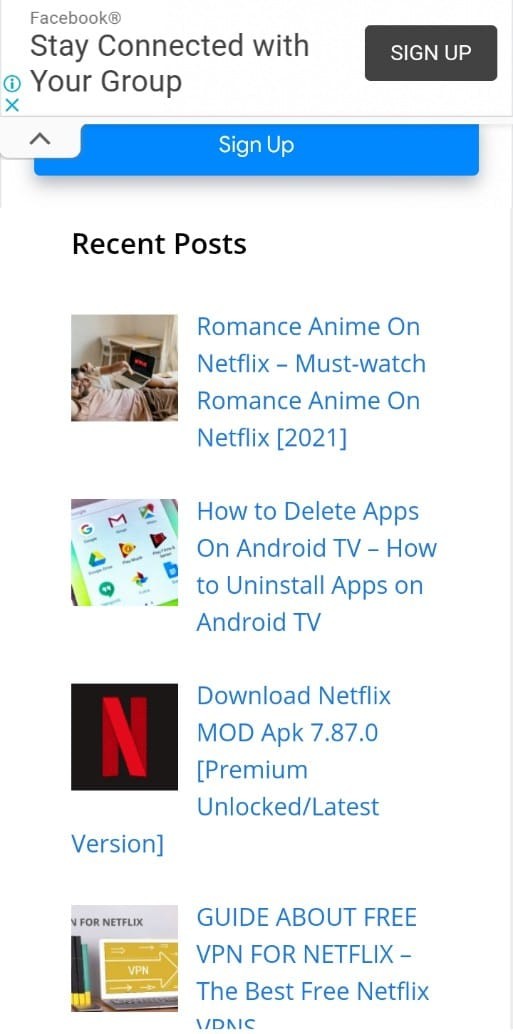The image displays a collection of elements aligned in a layout reminiscent of a Facebook interface, replete with promotional content and instructional images related to different digital services and tools. At the top, the familiar "Facebook" logo is accompanied by a subtle gray registered trademark symbol. Below this masthead, bold black text on a white background urges users to "Stay connected with your group." To the right, accessible call-to-action buttons for "Sign Up," appear; one in white enclosed in a black square, and a more prominent version in white within a larger blue square. 

Adjacent to the sign-up prompts, a small white tab with an up arrow in black indicates expandable content. Below this, a header reads "Recent posts" in stark black text against a white backdrop. 

Below this header, a series of images cascade vertically, starting with an image evoking the clutter of a neglected bedroom. To the left, gray text advertises content: "Romance anime on Netflix," followed by the invitation, "Let's watch romance anime on Netflix 2021."

Next in the sequence is a cell phone screenshot offering instructions: "How to delete Android apps on Android TV" and "How to install apps on Android TV." This is closely followed by the striking red Netflix logo set against a black background. Adjacent gray text promotes a downloadable Netflix mod pack, version 7.87.0, with features like "Premium unlocked, latest version."

Further down, an image of a laptop screen displays the term "VPN" in vivid yellow and white text. Accompanying gray text reads "Guide about free VPN for Netflix," though the phrase "the best free Netflix VPNs" gets truncated at the bottom.

A thin gray line outlines the left edge of the image, providing a clean aesthetic border to the content-laden visual.

In summary, the image serves as a multifaceted visual repository, encompassing promotional material, guides, and calls-to-action for a diverse array of digital products and services, all presented against the familiar visual framework of the Facebook platform.